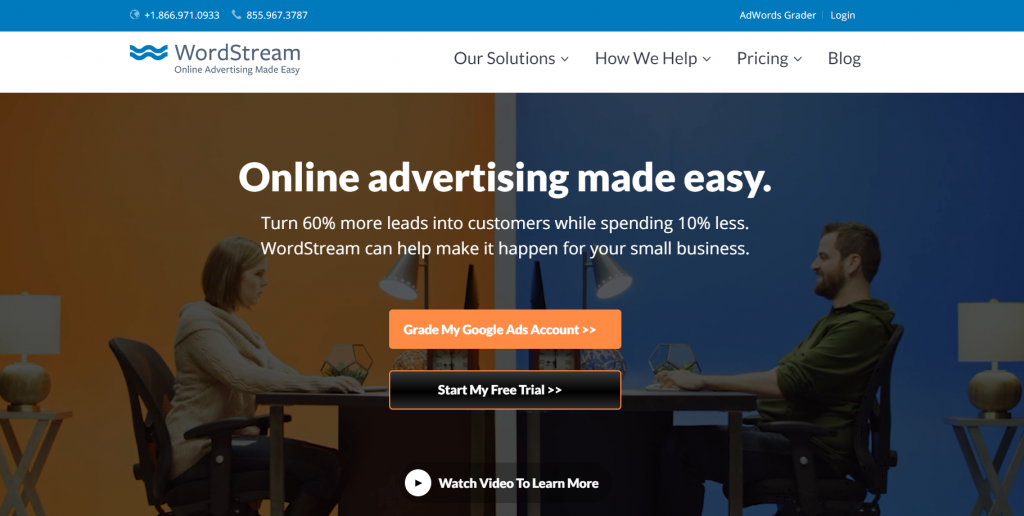The landing page of the WordStream website, titled "WordStream Online Advertising Made Easy," conveys a clear and user-friendly first impression. 

Starting from the upper left-hand side of the page, the company's name, "WordStream Online Advertising Made Easy," is prominently displayed. To the left, contact numbers are provided: 1-866-971-0933 and 855-967-3787.

In the center of the top navigation bar, key menu items are listed: "WordStream," "Our Solutions," "How We Help," "Pricing," and "Blog." Above this menu, on the same line as the contact numbers, additional links are available: "AdWords," "Creator," and "Login."

Beneath the navigation bar, a central photo emphasizes the headline "Online Advertising Made Easy." The accompanying text promises, "Turn 60% more leads into customers while spending 10% less. WordStream can help make it happen for your small business."

Below the photo and text, calls to action are presented in distinct colored boxes: an orange box with "Create my Google Ads account," a black box with "Start my free trial," and a link to "Watch video to learn more."